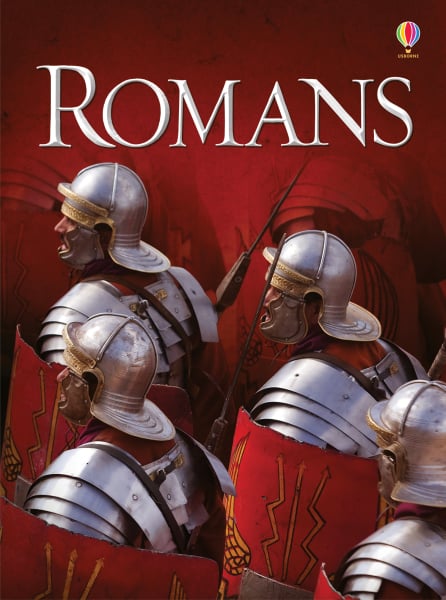The image features a striking red background with large white text at the top that reads "Romans." In the top right corner, there's a small, multicolored hot air balloon logo. The main focus is a close-up of four Roman legionaries clad in full battle gear, including silver metal helmets that have a flat surface extending along the back, with golden or brass accents and a cross design running from ear to ear and front to back. They are holding red shields adorned with yellow designs that resemble two lightning strikes and a central straight line. The shield also features wing-like patterns on the left side. The legionaries are shown from the head and shoulders down, and their bodies are obscured by their protective shields.